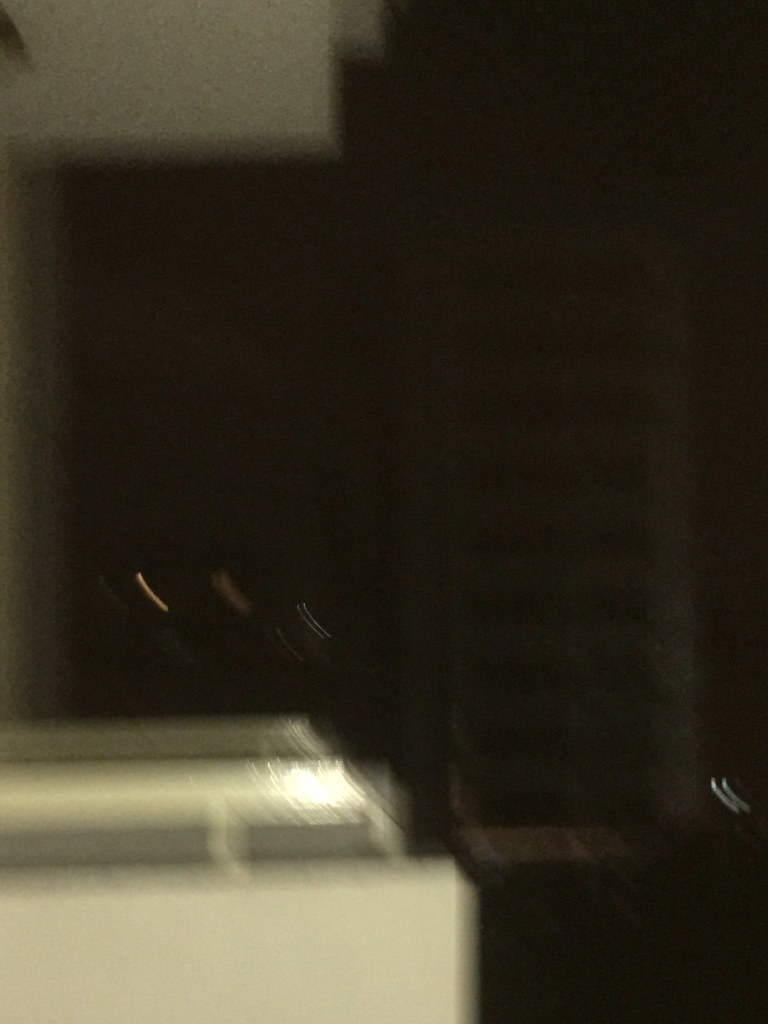A highly blurred and out-of-focus photo, likely taken accidentally, dominates the frame with a large expanse of darkness. In the lower-left corner, a brighter section reveals the possibly illuminated intersection of a wall and ceiling. The bright blur in this area suggests the presence of a light source. Above this, within the dark zone, three lighter streaks are visible, possibly overexposed and blurry distant lights. At the top of the image, a white area in the top-left corner could indicate another segment of the wall. Overall, the image seems to depict a very unclear and indiscernible view, potentially through a window.